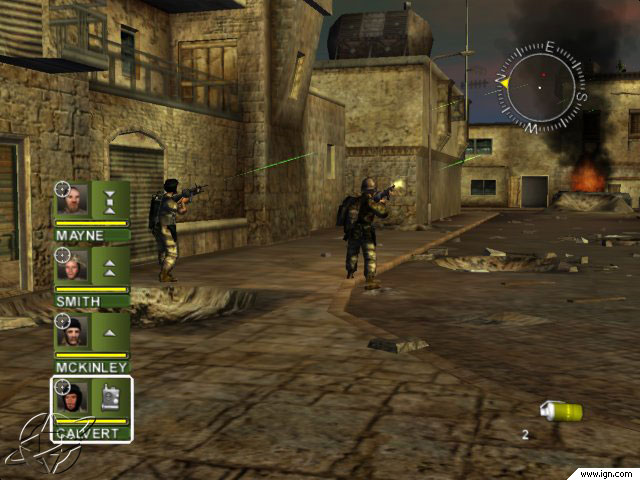A screenshot from an early 2000s military shooting video game, set in a war-torn Middle Eastern town. The game's graphics reflect the era's technology, presenting a gritty and intense battlefield environment. On the left side of the screen, four characters are listed: Maine, Smith, McKinley, and Calvert. Two of the military members are depicted wielding rifles equipped with green laser sights, highlighting their readiness for combat. The overall scene captures the chaotic and perilous atmosphere of the war zone. A watermark at the bottom of the image reads "www.IGN.com," indicating the source of the screenshot.